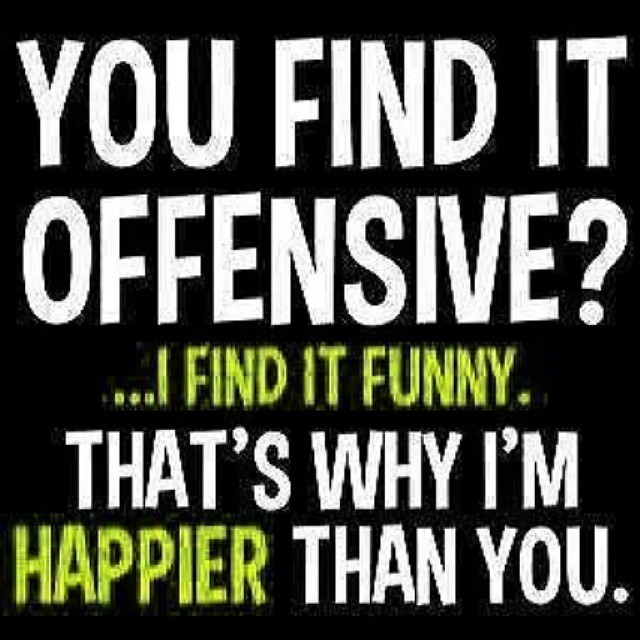This is a square meme graphic with a completely black background and bold block text in white and yellow. The text is arranged into five lines. The first line in large white letters reads, "You find it offensive?" The second line in yellow, slightly smaller, says, "...I find it funny." The third and fourth lines switch back to white and read, "That's why I'm" with the fifth line in bright yellow stating, "happier" followed by "than you" in white. The overall message of the image is, "You find it offensive? ...I find it funny. That's why I'm happier than you." There are no other design elements, photos, or additional text on this graphic.